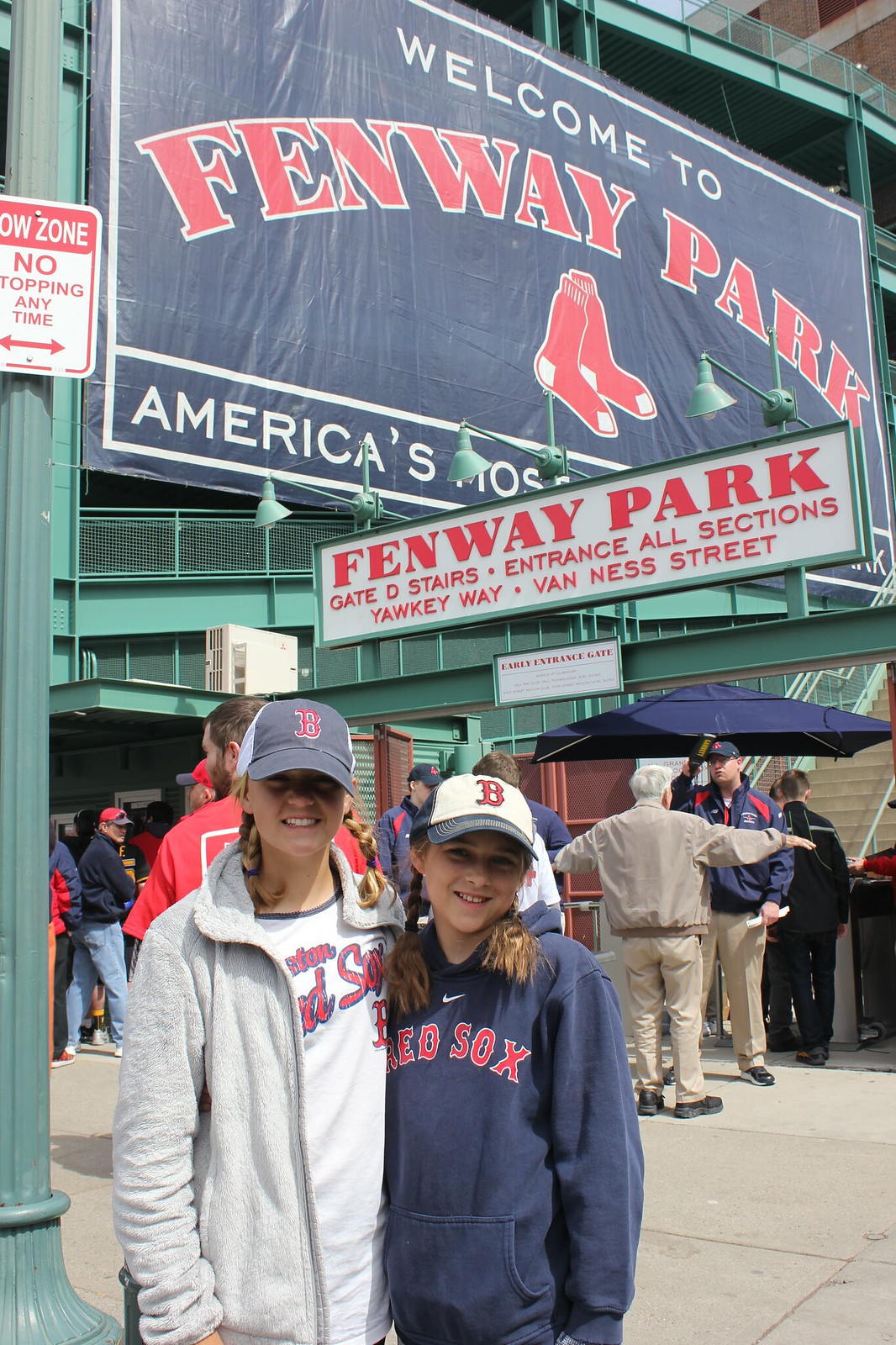The image depicts two young girls standing in front of the entrance to Fenway Park, facing the camera. Both girls are wearing Boston Red Sox paraphernalia, including baseball caps with the Boston logo. The girl on the left is dressed in a gray zip-up sweatshirt over a white shirt with "Boston Red Sox" in red lettering. The girl on the right has braided pigtails and is wearing a blue hoodie with the Red Sox logo and a Nike logo at the neck. Behind them, a bustling crowd is visible, including a man being scanned by security. Prominently displayed above the crowd is a large navy sign with "Welcome to Fenway Park" in white and red letters, accompanied by the Boston Red Sox logo. Another sign below reads "Fenway Park, Gate D stairs, entrance all sections, Yawkey Way, Van Ness Street." The green structure and the vibrant scene suggest a lively atmosphere typical of a game day.